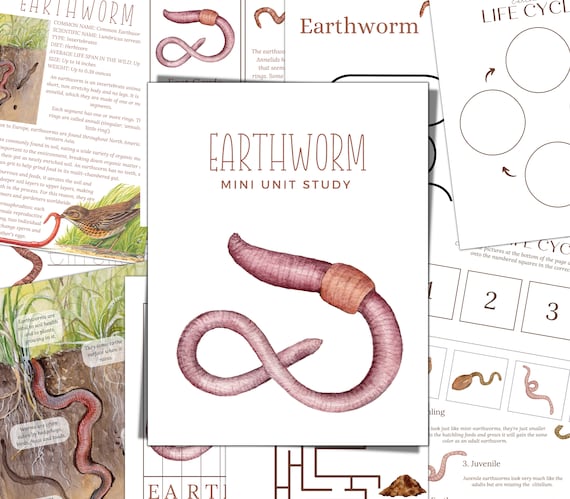The color image displays a collection of educational materials focused on earthworms that are spread across a surface. Central to the image is the cover of a mini-unit study guide, which is white and features a pink, figure-eight-shaped earthworm illustration towards the bottom. The cover has the title "Earthworm" in bold brown text and "Mini Unit Study" written beneath it. Surrounding the cover are scattered pages from the study, depicting various detailed illustrations and activities related to earthworms. These include images of a bird eating a worm, a worm burrowing into the ground with a cross-section view showing grass above the soil, and additional illustrations and worksheets towards the right side. Key educational activities visible on these pages include life cycle stages marked with numbers and corresponding images, likely for matching exercises, and other interactive elements such as a maze. The materials collectively provide a comprehensive, visual approach typical of a textbook or study guide intended for learning about the life and behavior of earthworms.